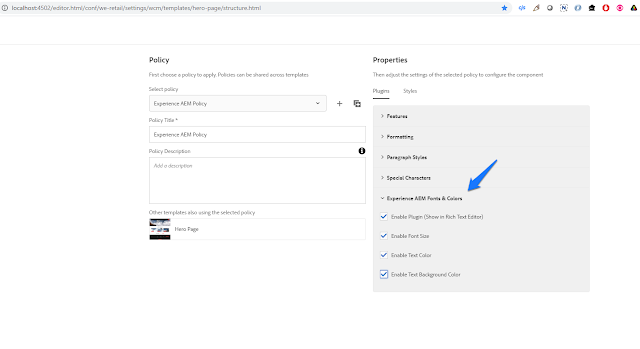Screenshot of a web page with a white background. The top browser bar displays the URL: `localhost:4502/editor.html/conf/we/retail/settings/scm/templates/hero-page/structure.html`, indicating the page being edited. To the far right of the bar, a small blue five-pointed star signifies that this page has been bookmarked. Adjacent to the star, there are approximately seven small icons, though the details of these icons are not clearly visible.

Below the browser bar, the main content area of the web page is divided into sections. On the left side, the text reads:

"**Policy**
First, choose a policy to apply. Policies can be shared across templates."

Beneath this text is a dropdown menu labeled "Select Policy," which currently displays the option "Experience A Policy." To the right of the dropdown menu are two icons: a plus sign and a share icon.

Further down, the page has the following heading:

"**Policy Title**
Experience A Policy"

The layout and instructions suggest that this section is used to manage and apply different policies to web templates.